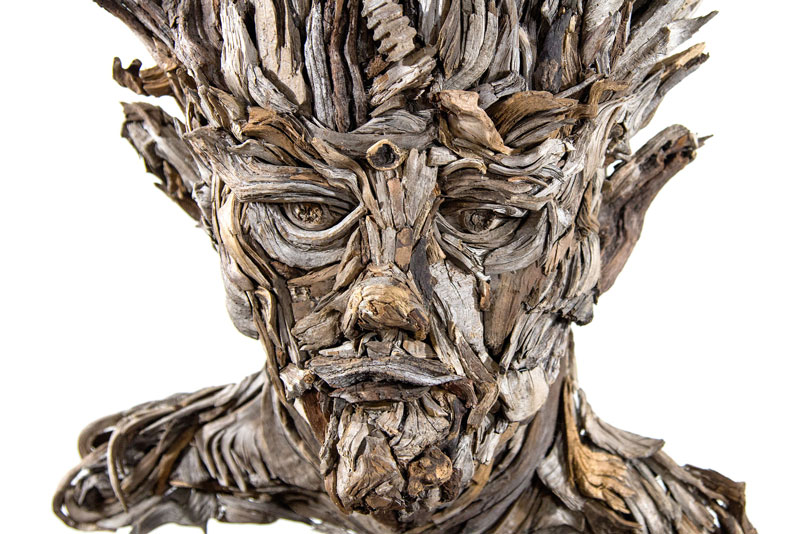The image showcases a highly detailed sculpture of a man's head, constructed meticulously from various pieces of tree bark, roots, and dried wood parts. The craftsmanship highlights a range of textures and colors, including beige, brown, gray, and light gray tones. The man's facial features—eyes, nose, lips, and ears—are clearly defined, with the eyes appearing greenish-brown and detailed enough to show the whites. His hair is styled to stick straight up and appears quite long. The sculpture also includes a goatee-like beard and prominently protruding lips made from sticks. Notably, there is a jewel-like round object positioned between his eyes, adding an element of intrigue. The ears jut out noticeably from either side of his head, and the shoulders, although just the tops, are visible, adding to the realism. The background of the photograph is a stark white, providing no additional context for the size of the sculpture but offering a close-up, detailed view of this imaginative piece of art.